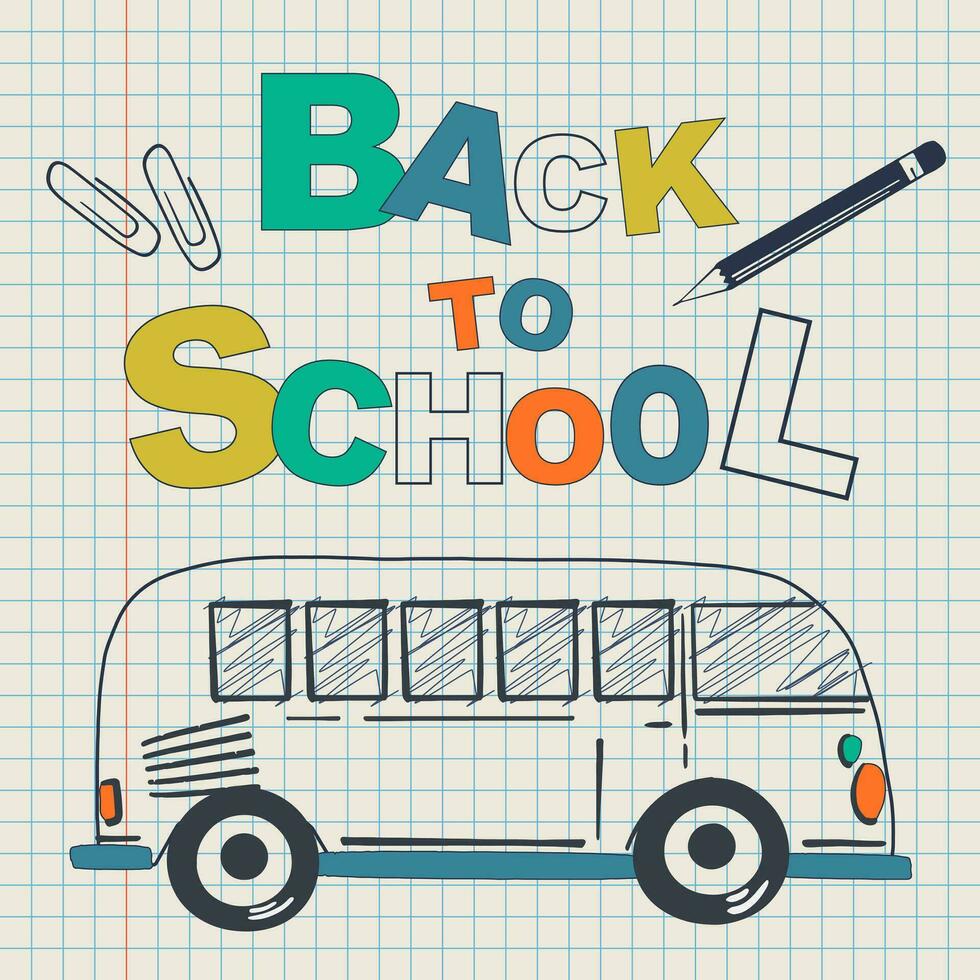This poster, likely seen inside a store, vividly advertises the back-to-school season with an illustration on loose-leaf grid paper. The background has the characteristic blue grid lines and a vertical red margin line, typical of notebook paper. Prominently displayed in simple block letters at the top are the words "BACK TO SCHOOL," each letter meticulously colored and uncolored as follows: the "B" is green, "A" is blue, "C" remains plain white, "K" is yellow, "T" in "TO" is orange, the "O" is blue, while in "SCHOOL," "S" is yellow, "C" is green or teal, "H" is plain, the first "O" is orange, the second "O" is blue, and "L" remains unfinished.

Below the text, there is a sketch of a bus that seems partially colored. The main body of the bus is left white, blending with the paper, but it features orange headlights and taillights, a green turn signal, a blue bumper, black tires, and black wheel centers. The bus, resembling more of a minivan or a vintage Volkswagen van, is accompanied by additional drawings: two black and white paper clips and a profile of a pencil with a black eraser in the top left corner. The entire design exudes a hand-drawn, whimsical feel, perfectly capturing the essence of going back to school.